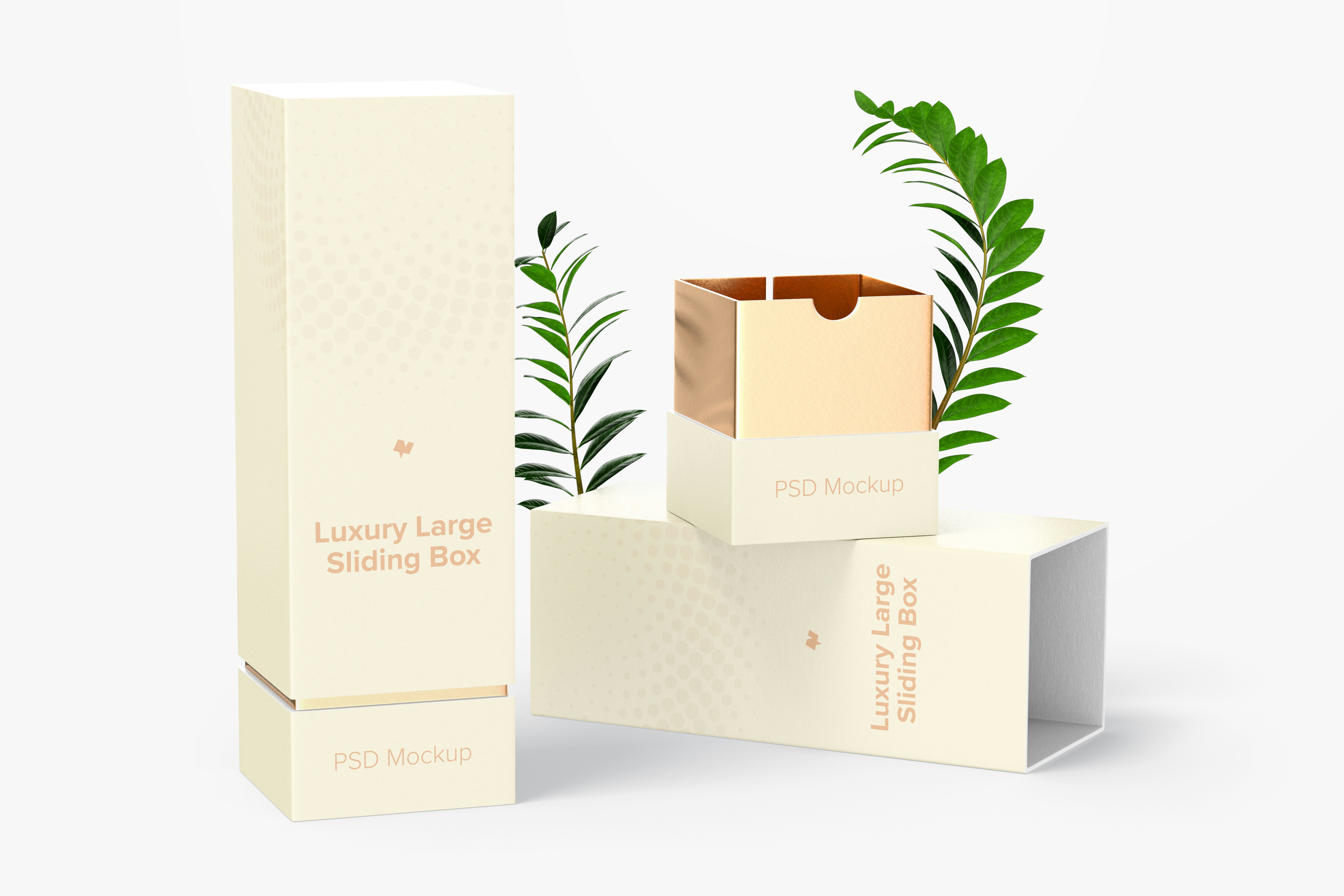The image features a meticulously arranged product mock-up set against a pure white background. Central to the composition is a tall, off-white, cream-colored box labeled "Luxury Large Sliding Box" with dark gold lettering. This box stands upright with its top and bottom separable by sliding. To the right of this upright box, there is another identical box, positioned horizontally. On top of this horizontally oriented box sits an open, smaller, square box that is partially pinkish at the bottom and transitions to a gold color at the top, bearing the label "PSD Mock-Up." The top of this smaller box, also labeled "PSD Mock-Up," is detached and placed beneath the upright box. Behind the boxes, two green fern branches are prominently displayed, adding a touch of nature to the otherwise minimalist scene. The entire setup casts subtle shadows, enhancing the realism of the mock-up.